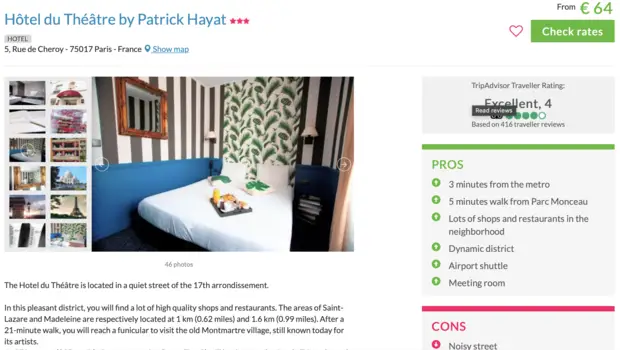The image prominently displays an advertisement for the Hotel du Théâtre by Patrick Hyatt. It provides the address as Rue de Cheroy, Paris, France. The advertisement highlights several images, including a detailed shot of a bedroom, alongside a grid displaying twelve smaller images—six in a left column and six in a right column. The text describes the hotel’s location in a quiet street of the 17th arrondissement, emphasizing the district's abundance of high-quality shops and restaurants. It also mentions the proximity of notable areas, with Saint-Lazare and Madeleine situated approximately 1 kilometer and 1.6 kilometers away respectively. On the right side of the advertisement, there is pricing information starting from £64 with an option to check rates by clicking a green box. At the bottom, there is a section listing the pros and cons of the hotel, with cons highlighted in red.